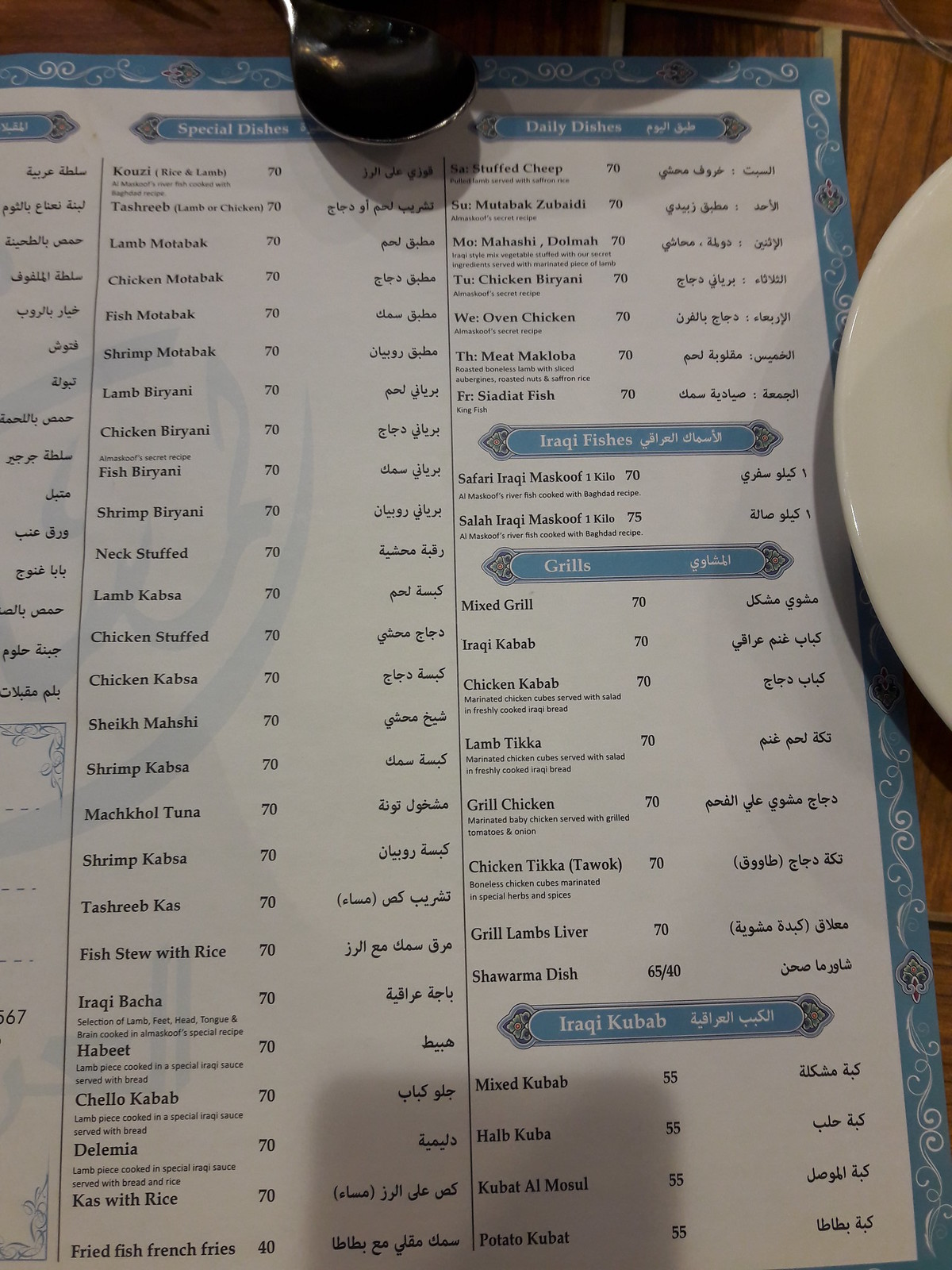This photograph captures the essence of an Iraqi restaurant's menu, prominently displayed on what appears to be a brown wooden dining table. Dominating almost the entirety of the frame, the menu is adorned with a blue border embellished by white swirly lines. At the top of the menu, a silver soup spoon is placed, adding a touch of metallic elegance. To the right edge of the menu, the rim of a white ceramic plate is barely visible, hinting at the dining experience awaiting guests.

The menu itself features a subtle, off-white blue background with the restaurant’s logo faintly superimposed in the center. In the middle section of the menu, there is a list of special dishes priced at 70 units of an unspecified currency. The text is bilingual, with the names of the menu items presented in English on the left and their Arabic counterparts shown alongside the prices on the right.

On the right side of the photograph, other sections of the menu are visible, indicating categories such as daily dishes, Iraqi fishes, grills, and Iraqi kebabs. Each section header is also presented in both English and Arabic, maintaining a consistent bilingual format. Unfortunately, the leftmost portion of the menu is cut off in the photo, leaving some sections unreadable.

This detailed capture elegantly combines elements of cultural cuisine, language, and meticulous design, providing an inviting glimpse into the dining experience offered at this establishment.